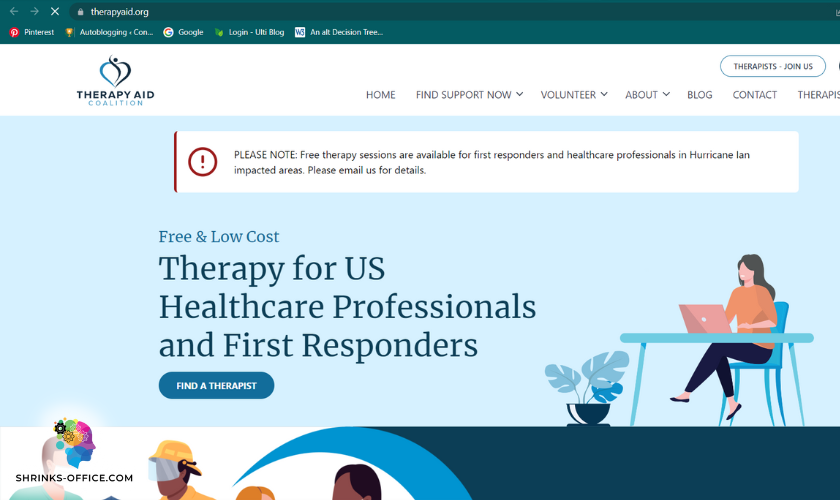In this image, we are presented with a screenshot of a website designed to assist individuals in finding therapy services. The URL "therapyaid.org" is prominently displayed at the top within a green header. The website showcased belongs to the "Therapy Aid Coalition" and offers several navigation options on the right side including: Home, Find Support Now, Volunteer, About, Blog, Contact, and Therapists.

A notable feature of the website is a pop-up message alerting visitors that free therapy sessions are available specifically for first responders and healthcare professionals affected by Hurricane Ian, along with a prompt to email for further details.

The main body of the site features a light blue background with the text, "Free and low-cost therapy for U.S. healthcare professionals and first responders." Directly below this, there is a clickable button labeled "Find a Therapist."

To the far right of the page, there is an illustrative graphic depicting a woman with long dark hair, wearing an orange shirt and black pants, sitting at a blue table in a blue chair, engaged with a laptop. The overall layout and design of the website emphasize its focus on providing accessible mental health support to those in need.